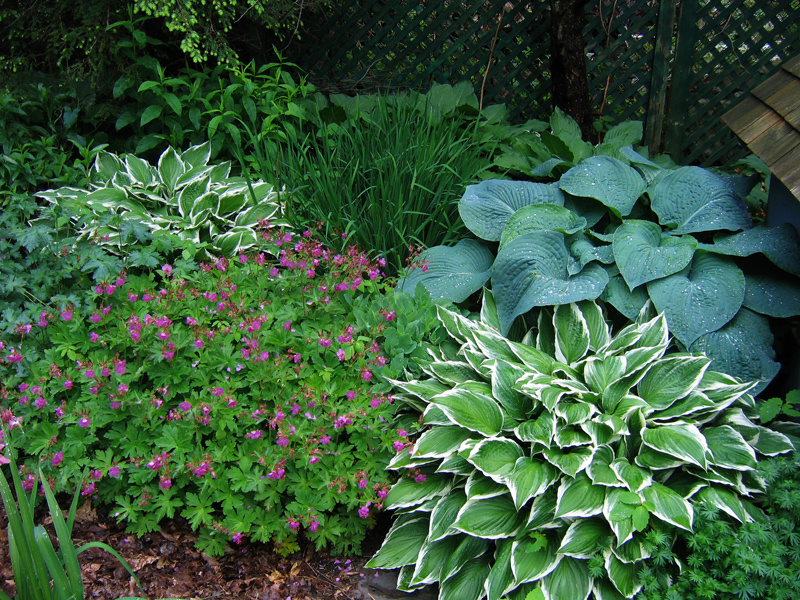The photograph captures a vibrant garden plot brimming with diverse and healthy foliage. Dominating the scene are several varieties of hostas, including two clusters of medium green leaves edged in white and another cluster of bluish-green leaves. Among these are an assortment of other plants, each contributing to the garden's lush diversity with their unique leaf shapes and sizes—ranging from large to tiny and narrow. The garden's health is evident in the bright, fresh appearance of the leaves. At the bottom of the image, brown soil sprinkled with dried leaves is visible, along with patches of small grass. Notably, in the bottom left corner, there is a plant adorned with tiny purple flowers. In the background, a green lattice fence provides a quaint backdrop, and to the right, there is a hint of a shingle roof near the ground, possibly indicating a dog house. Adding to the visual interest, a small bush with red, bleeding hearts flowers stands out amid some grass and occasional weeds growing along the lattice.